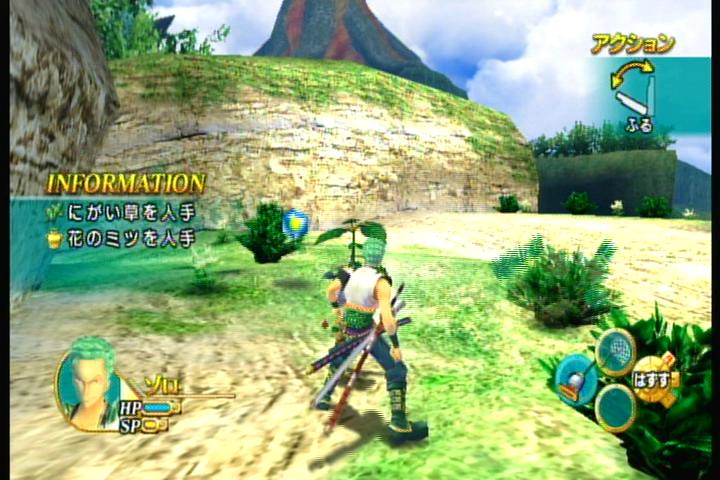This screenshot depicts a third-person Japanese video game with old, blocky visuals. The central character, identifiable by his green hair and green mesh helmet, is a warrior clad in blue pants, combat boots, a white tank top, a gray vest, and wristbands. He carries multiple swords at his right hip. The scenery is set outdoors, featuring a vibrant landscape with high cliffs, a volcano with gray and orange hues, and a variety of greenery including trees, bushes, and grassy areas. The sky is blue, dotted with white, puffy clouds. The lower left corner of the screen displays the character's hit points (HP), special attacks (SP), and a circular image of the character's face. An information section with yellow or gold lettering and additional Japanese text is also visible on the left. Over on the right, partially obscured by bushes, are icons that appear to represent various weapons, such as a bomb and a landmine, with associated numbers or Japanese characters. The character is navigating through a valley, with a rocky, multicolored hill and a ledge in the background.